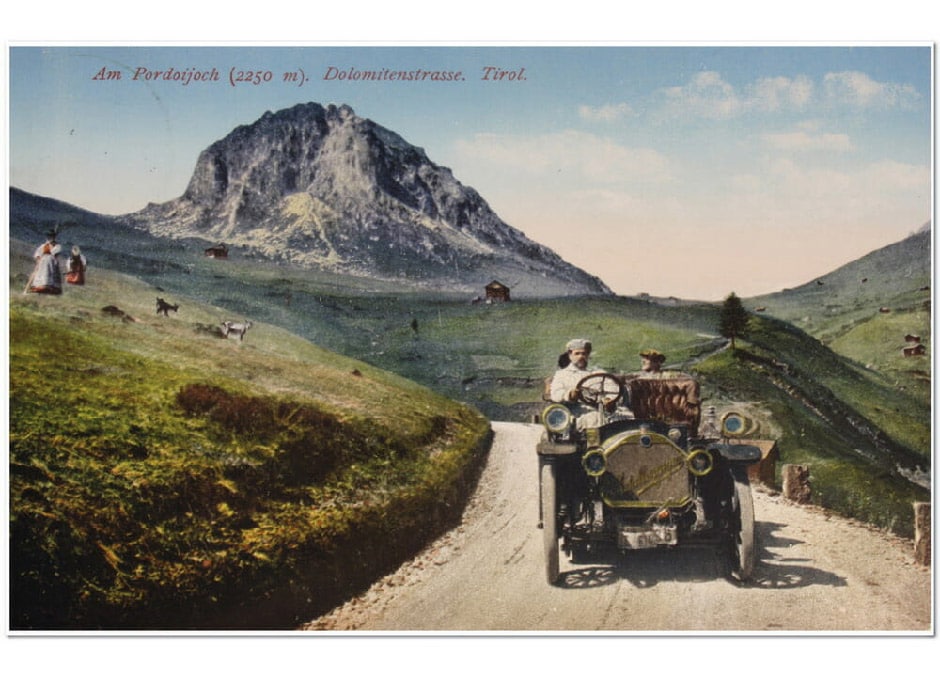This vibrant and meticulously detailed painting captures a picturesque scene of a man driving a vintage car from what appears to be the 1920s. The car, reminiscent of early automotive designs, possibly a Rolls Royce though shaped like a Model T, comes with an open top, distinctive wooden wheels, and a prominent radiator at the front. The driver is alone in the front seat, with a passenger seated in the back seat on the passenger side, while the passenger seat remains empty. 

The car travels along a gravel road winding through a mountainous region, the majestic peaks forming a breathtaking backdrop. The setting is rendered in bright, natural daylight, with a clear blue sky dotted with fluffy white clouds. Surrounding the road, green terrain spreads outwards, populated sporadically with women on the hills to the left and various animals—primarily lambs and goats—gathered near a few rustic wooden buildings. In the top left corner of the image, there are some inscriptions written in an undecipherable language, adding an element of intrigue to the scene. The painting exudes a sense of time, place, and serenity, capturing a moment from a bygone era with exceptional clarity and vividness.